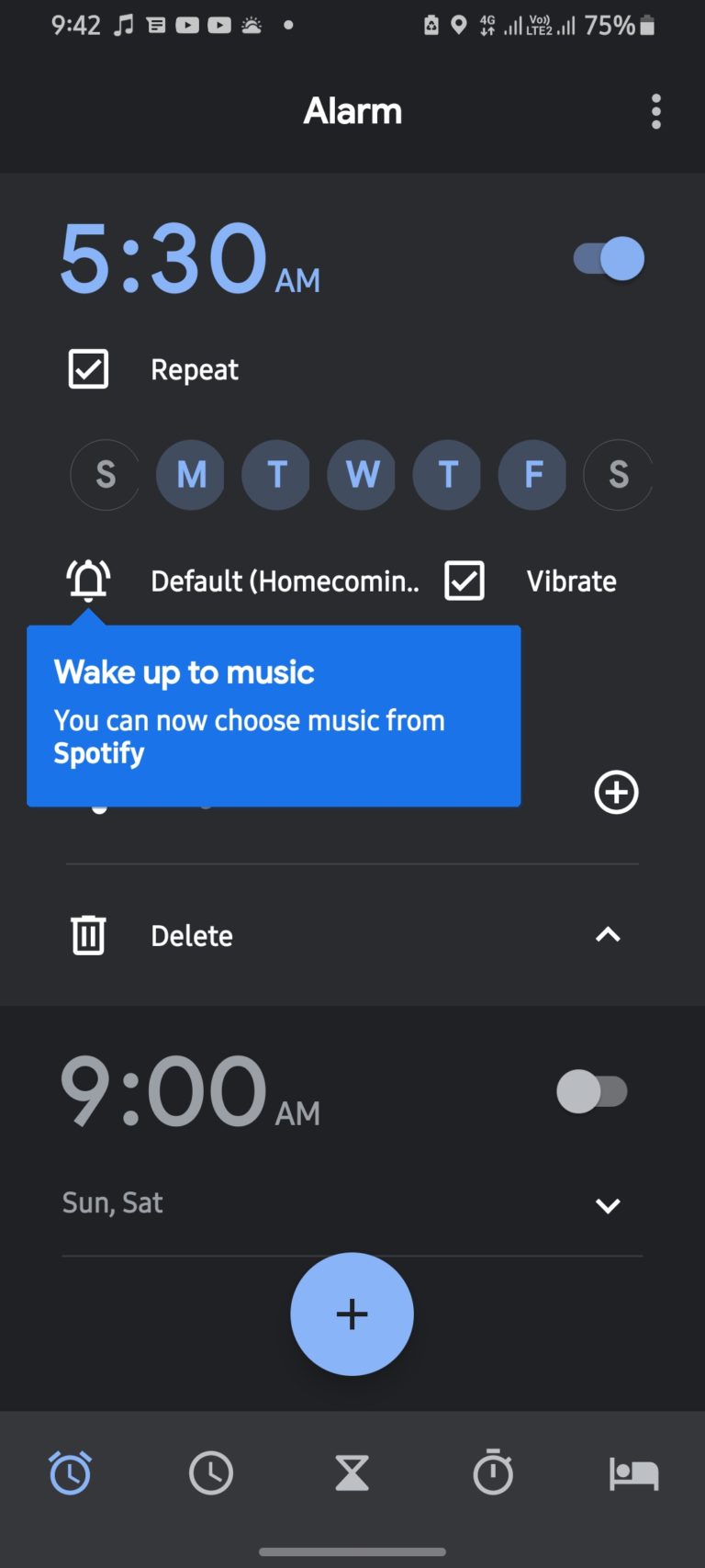*Screenshot of the Alarm Settings*

The image is a screenshot displaying the alarm settings on a smartphone with a black background adorned with blue and white text. The time shown on the screenshot is 9:42 PM. Here are the key elements detailed in the image:

- **Alarm Details:**
  - The alarm is set for 5:30 AM, highlighted in blue text against the black background.
  - It is turned on and set to repeat every weekday (Monday through Friday) but not on weekends (Saturday and Sunday).
  - The alarm is configured with a default green tone named "Homecoming."
  - The wake-up music feature is enabled, allowing the user to choose a song from Spotify.
  - The alarm is also set to vibrate.
  - Options available include deleting the alarm and adding more alarm times.

- **Notifications and Widgets:**
  - There are unread text messages indicated.
  - Two pending YouTube videos are awaiting the user's attention.
  - The weather widget is active, providing current weather information.

- **Device Status:**
  - The phone is in power-saving mode.
  - Google Location service is turned on.
  - The device has full 4G LTE signal strength.
  - Volume levels are set to maximum.
  - The phone battery is at 75%.

- **Additional Features:**
  - There are various mode buttons at the bottom of the screen, including sleep mode, timer mode, and others.
  - The alarm for 9:00 AM on Saturday and Sunday is currently set to off.

Overall, the screenshot captures a comprehensive view of the user's alarm settings and offers insights into their phone's status and additional configurations.